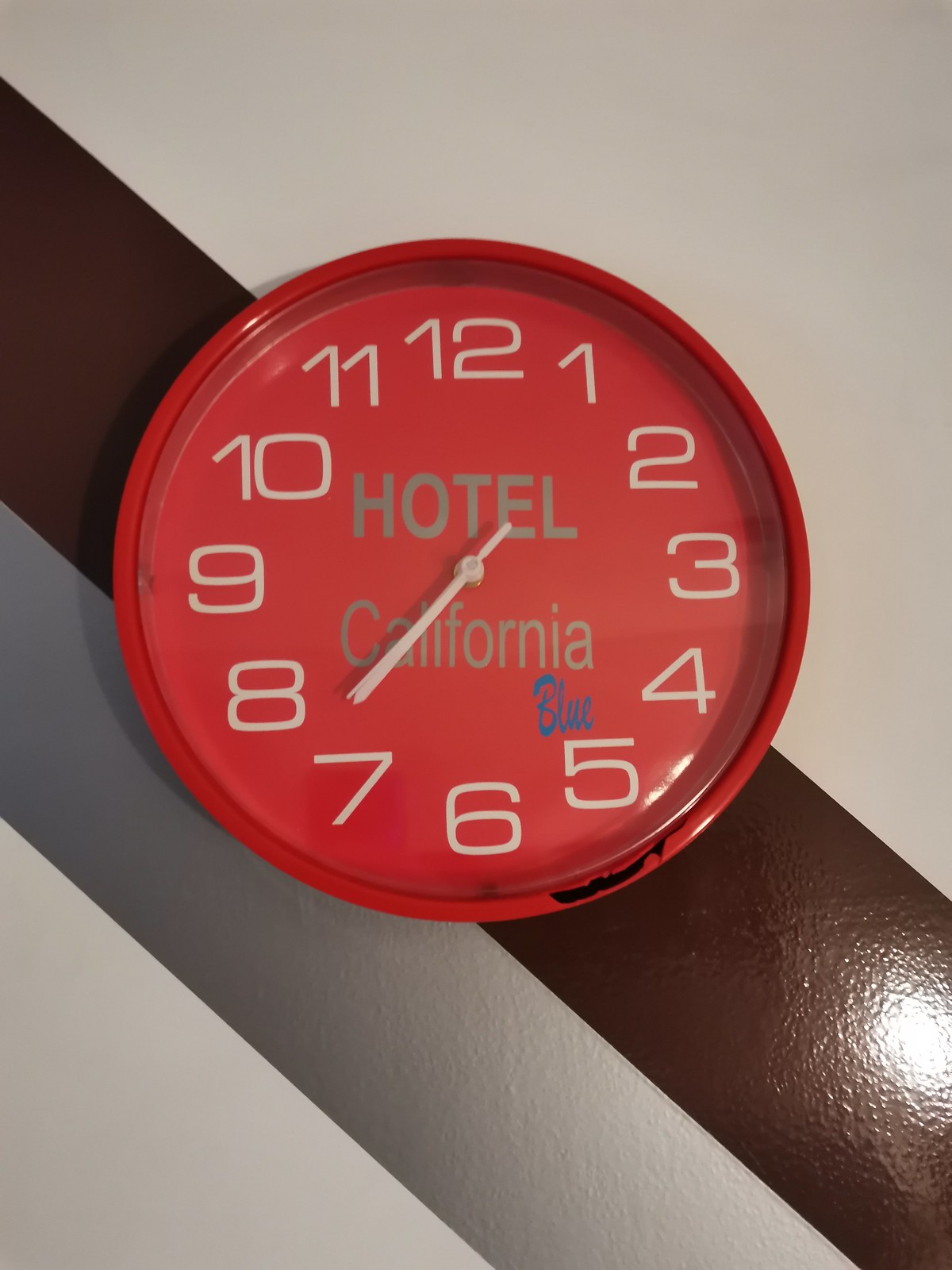This detailed photograph showcases a striking red analog clock, fashioned from what appears to be a shiny serving tray, corroded at the bottom revealing patches of black. The round clock face prominently features white standard numbers and two white hands indicating the time as approximately 22 minutes to 8. At the center of the clock face, the words "Hotel California" are inscribed in silver, and just below "California," on the bottom right, the word "blue" is written in blue script. The clock is mounted on a wall displaying distinct background stripes: a shiny brown stripe running diagonally left to right, intersecting with a darker gray stripe, and a white section on the bottom left, all set against a gray backdrop, adding depth and contrast to the sharp, detailed image.